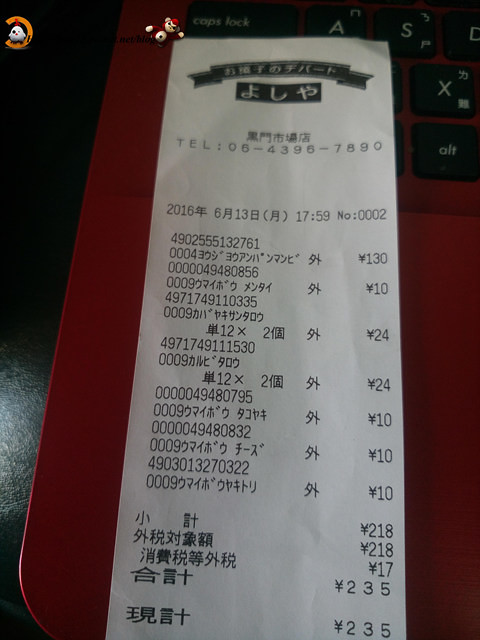A crisp, long white receipt, printed in either Chinese or Japanese, rests perfectly aligned on a sleek, dark calculator or cash register. At the very top of the receipt, a black stripe boldly dons the name of the establishment in striking foreign characters, immediately capturing attention. Below this, another black rectangle features white lettering in the same language, perhaps specifying additional important information. Further down, a clearly displayed telephone number suggests where the establishment might be contacted. The bulk of the receipt continues with an itemized list of purchased items, each carefully detailed alongside their corresponding prices, offering a clear and organized summary of the transaction.